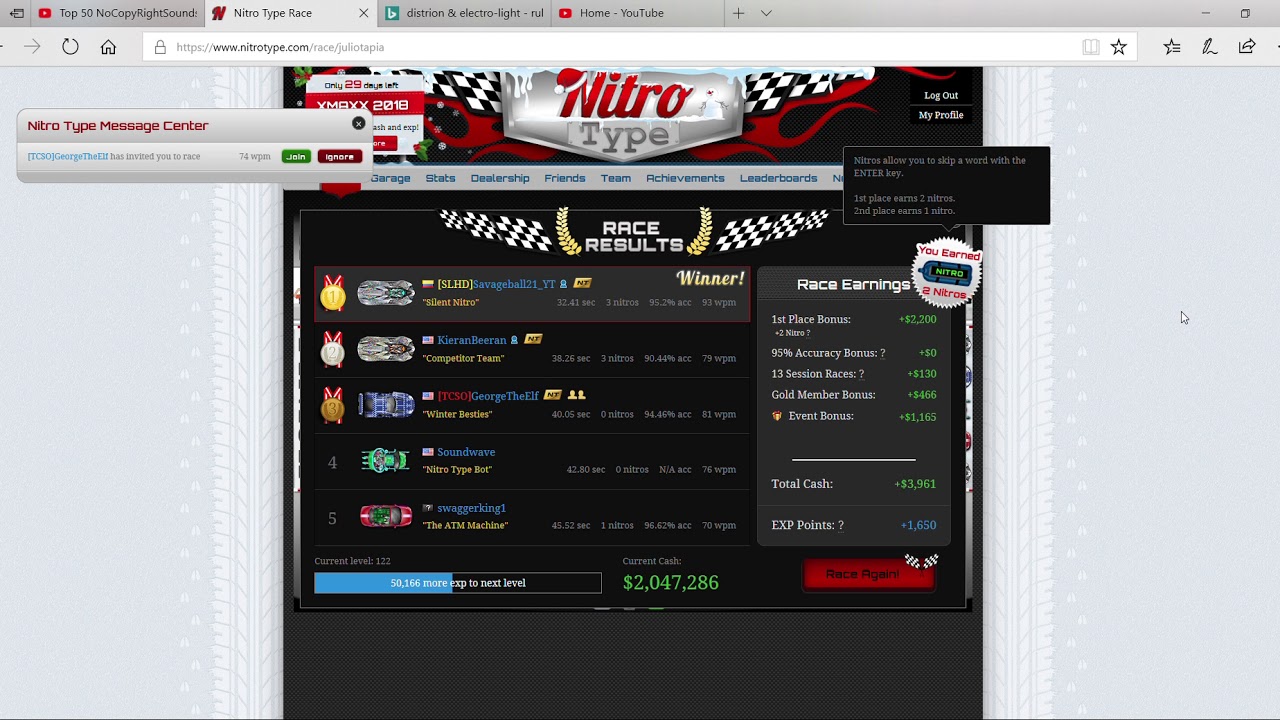**Caption:**

A comprehensive screenshot of the Nitro Type website is displayed. At the top, a festive header showcases the Nitro Type logo, with "Nitro" in vivid red and "Type" in muted gray, set within a shiny, gray, rectangular shield design. The header is adorned with snow on top, adding a wintery touch, and a Santa Claus hat perched above the “N” in Nitro highlights the seasonal theme. The outer edges of the shield feature checkered black and red racer stripes with red flame motifs beneath.

Below the header, a sleek gray navigation menu with bright blue letters offers various sections: Garage, Stats, Dealership, Friends, Team, Achievements, and Leaderboards. However, a black pop-up box partially conceals one of the menu items on the right. The pop-up explains, in gray font, that "Nitro allows you to add something with the Enter key," along with additional small text.

Underneath, a white circular badge announces, "You Earned," followed by "two Nitros" inside a blue rectangular box with the word "Nitro" in green. The main content area of the page has a black background with the title "Race Results" in white, flanked by checkered black and white flags. Below, a list of races is displayed, each accompanied by gold, silver, and bronze medals, and a race car icon on the left. The race names are in blue, with race descriptions in yellow quotation marks. Detailed race stats in gray font are on the bottom left of each race listing.

A detailed gray panel on the right side provides earnings information, titled "Race Earnings." This section delineates various bonuses: First Place Bonus ($2,200), a 95% Accuracy Bonus, Session Races Bonus (13 races - $130), Gold Member Bonus (approx. $166), and Everest Bonus ($1,163). The total cash amount is listed as $3,961. Below this, EXP points are noted as +1,650 in blue. 

At the screen's bottom left, a blue progress bar, about 40% filled, is overlaid with small, white text. Adjacent to this, current cash is detailed in gray as $2,047,286.

On the far right, a prominent red rectangular "Race Again?" button invites users to engage in another race. Flanking this button are black and white checkered racing flags, symbolizing the racing theme.

The top of the browser window, in gray, shows four open tabs: two YouTube tabs, a Nitro Type Race tab, and a Bing tab, reflecting a typical browsing session.